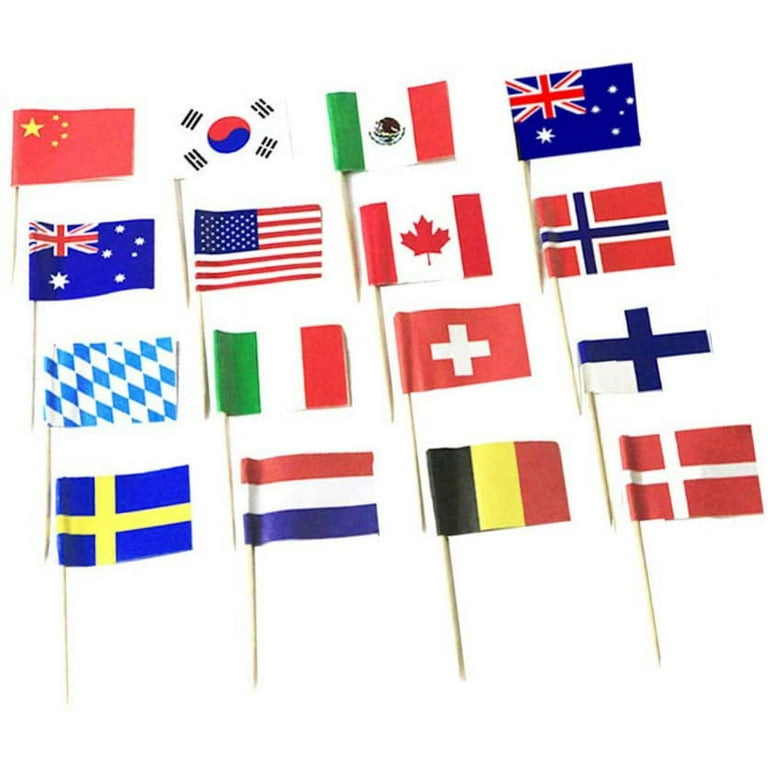The image depicts a 4x4 grid of miniature flags mounted on toothpicks, resulting in a total of 16 flags neatly arranged in rows. The flags showcase an array of national symbols from various countries around the world. In the top left, we see the flag of China, followed by the flags of South Korea, Mexico, and Australia. The second row includes the flags of the United States, Canada, and Norway, ending with a non-recognizable or fictional flag.

Continuing to the third row, there are flags of Italy, Switzerland, and Finland, followed by Sweden's flag with its distinct blue and yellow colors. The fourth and final row features the Netherlands' tricolor design, Belgium's black, yellow, and red, and Denmark's recognizable red flag with a white cross.

There is repetition and potential confusion regarding some flags, as the flag of Australia appears twice, with one possibly intended to represent New Zealand. Additionally, the UK flag is mentioned but seems to be in the array, along with descriptions like “red with a white cross” (Denmark or Switzerland), and "blue with a yellow cross" (Sweden). A vivid collection, this grid exemplifies global diversity through colorful emblems displayed on simple wooden toothpicks.